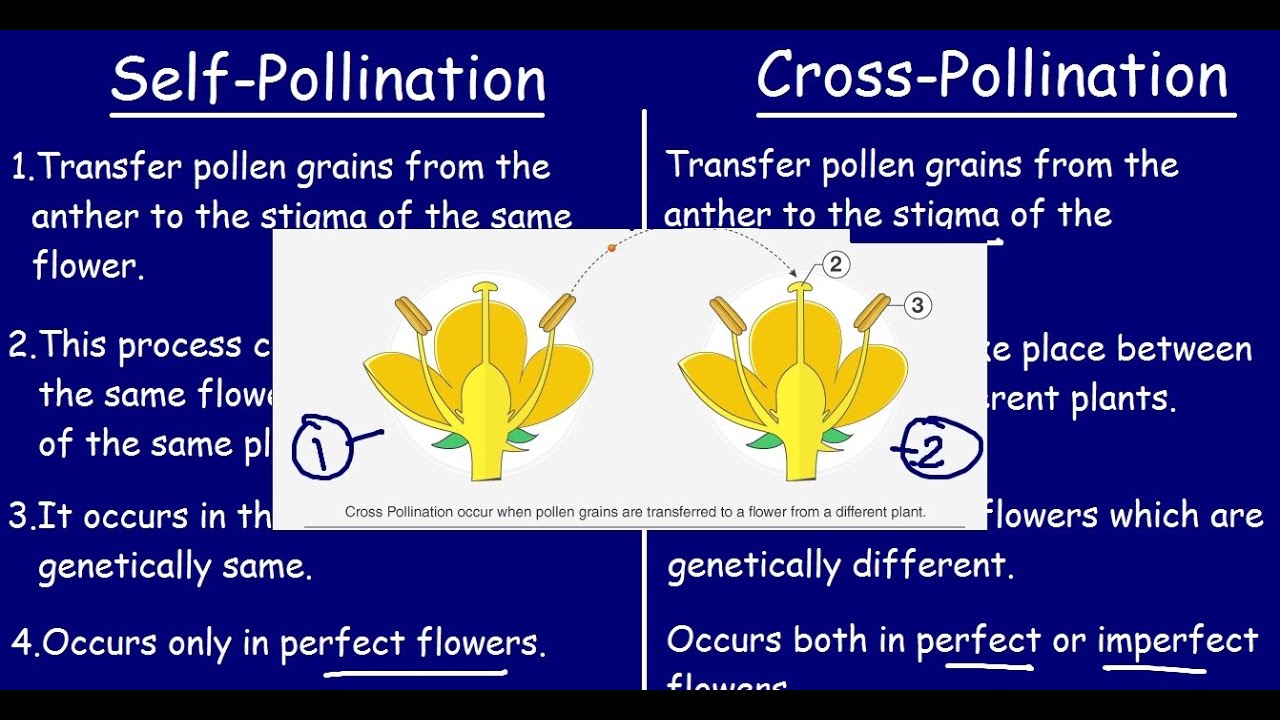The image features a diagram against a gradient blue background, transitioning to black at the top and bottom, detailing the processes of self-pollination and cross-pollination. The titles "Self-Pollination" and "Cross-Pollination" are prominently displayed in white Comic Sans font on either side of the image. Below the "Self-Pollination" heading, a numbered list highlights key points: 

1. Transfer pollen grains from the anther to the stigma of the same flower.
2. [Partially obscured text]
3. [Partially obscured text]
4. Occurs only in perfect flowers.

The "Cross-Pollination" section similarly notes the transfer of pollen grains from the anther to the stigma, with text cut off by overlapping white images. These images, presumed to represent self-pollination on the left and cross-pollination on the right, also feature yellow flowers. The diagram indicates that cross-pollination occurs in both perfect and imperfect flowers. The overall presentation, likely intended for an educational setting, resembles a slide one might see projected in a classroom.